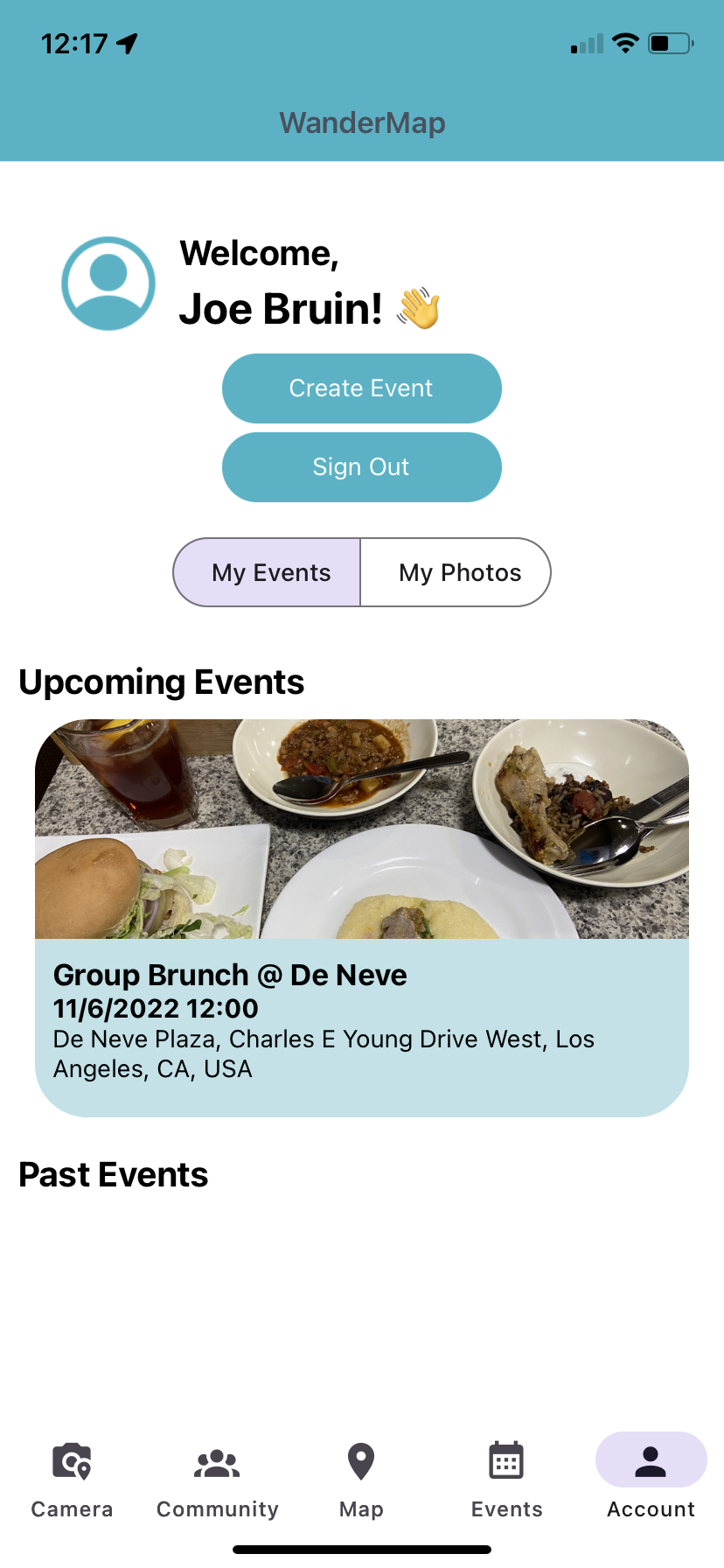The image displays a smartphone screen with the WandaMap application open. At the top left corner, the time is shown as 12:17, while the top right corner features three icons: a bedroom icon, a Wi-Fi icon, and a network signal icon, against a blue background.

In the center-bottom of the application, "WandaMap" is prominently written, identifying the app. Below this, on a white background, is a warm greeting "Welcome, Joe Bruin," accompanied by an orange waving hand emoji. Joe Bruin's profile picture is represented by a generic blue and white profile icon.

Beneath Joe Bruin's greeting, there are two horizontally-placed tabs with blue backgrounds and white text: "Create Event" and "Sign Out". Further down, there are two additional horizontally-aligned tabs: "My Photos" on the left, and "My Events" on the right, with "My Events" highlighted in purple, indicating it is currently selected.

Under the "My Events" tab, the section is titled "Upcoming Events," with the first event listed as "Group Brunch at Deneve," scheduled for November 6, 2022, at 12:00 PM, at Deneve Plaza, Charles A. Young Drive West, Los Angeles, CA, USA. This event is illustrated by an image featuring food on a white plate and in a white bowl, including a burger and a beverage.

The bottom of the screen displays the option "Past Event," and beneath that, there are navigation toggles for "Account" on the bottom right, and from right to left: "Events," "Map," "Community," and "Camera."